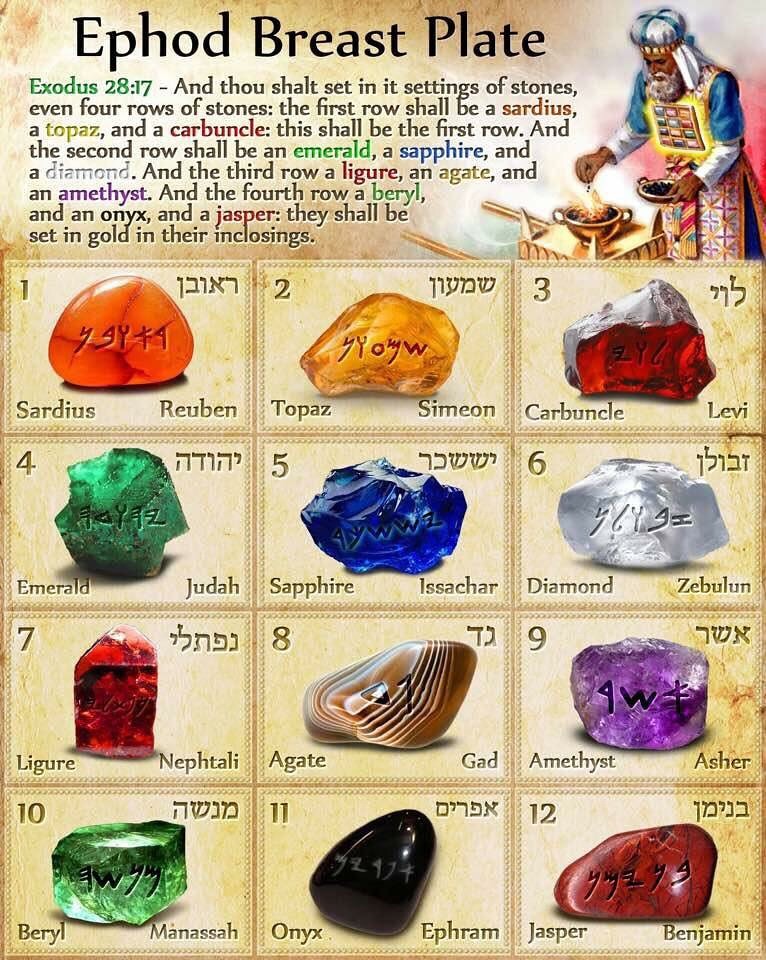This detailed poster, titled "Ephod Breastplate," features a semi-realistic illustration at the top right of a man in a blue robe with intricate gold and colorful designs, lighting a fire in a small golden pot. Below the title, there is a Bible quote from Exodus 28:17, which describes the settings of the stones. The central portion of the poster consists of a grid with three rows and four columns, showcasing twelve different gemstones. Each gem is depicted in vibrant colors ranging from orange, yellow, red, gray, blue, brown, black, to purple, and is accompanied by its name underneath. The stones listed include Sardius, Topaz, Carbuncle, Emerald, Sapphire, Diamond, Liger, Agate, Amethyst, Beryl, Onyx, and Jasper. Each gemstone is further associated with a name from the Bible, such as Reuben, Simeon, Levi, Judah, Zebulun, Nephthitely, Gad, Asher, Massa, Ephraim, and Benjamin, along with Hebrew inscriptions. The poster intricately aligns the gemstones in settings of gold, highlighting their biblical significance and historical context.